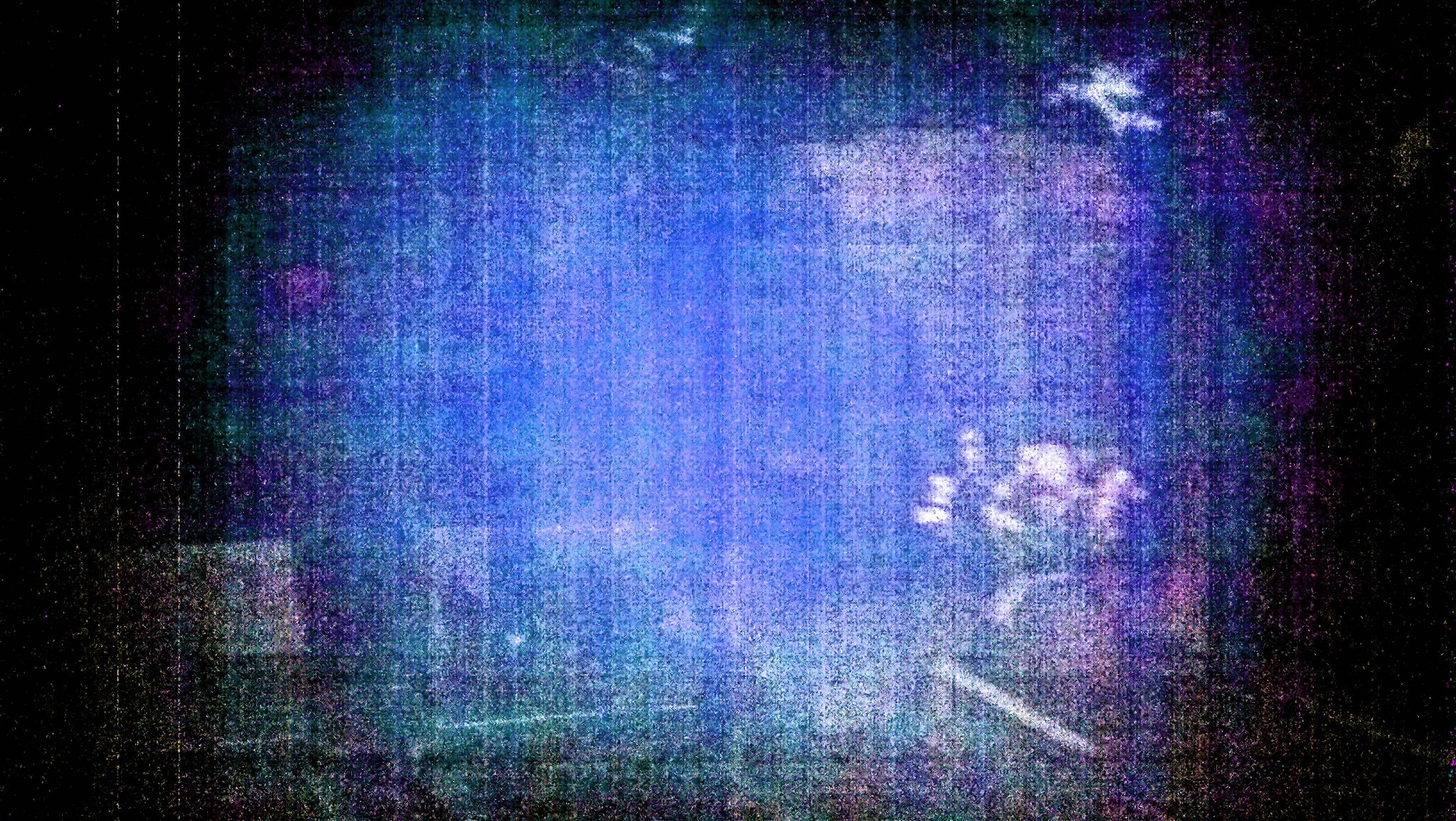This abstract painting features a low-resolution, pixelated texture that almost gives it a woven fabric appearance. Dominated by a royal blue hue, the painting is accentuated with streaks of light purple, violet, and lighter blue, creating a rich, dynamic background. At the bottom left and center, patches of green add depth, while a swatch of white mixed with gray occupies the right side, incorporating a distinct white line. The top right corner also contains a white splotch. Surrounding the blue central area are sections of black, interspersed with white streaks and purple highlights, contributing to a black denim-like effect. The combination of these elements and colors leaves the interpretation of the painting up to the viewer, with some perceiving elements like a skier or box shapes within the composition.